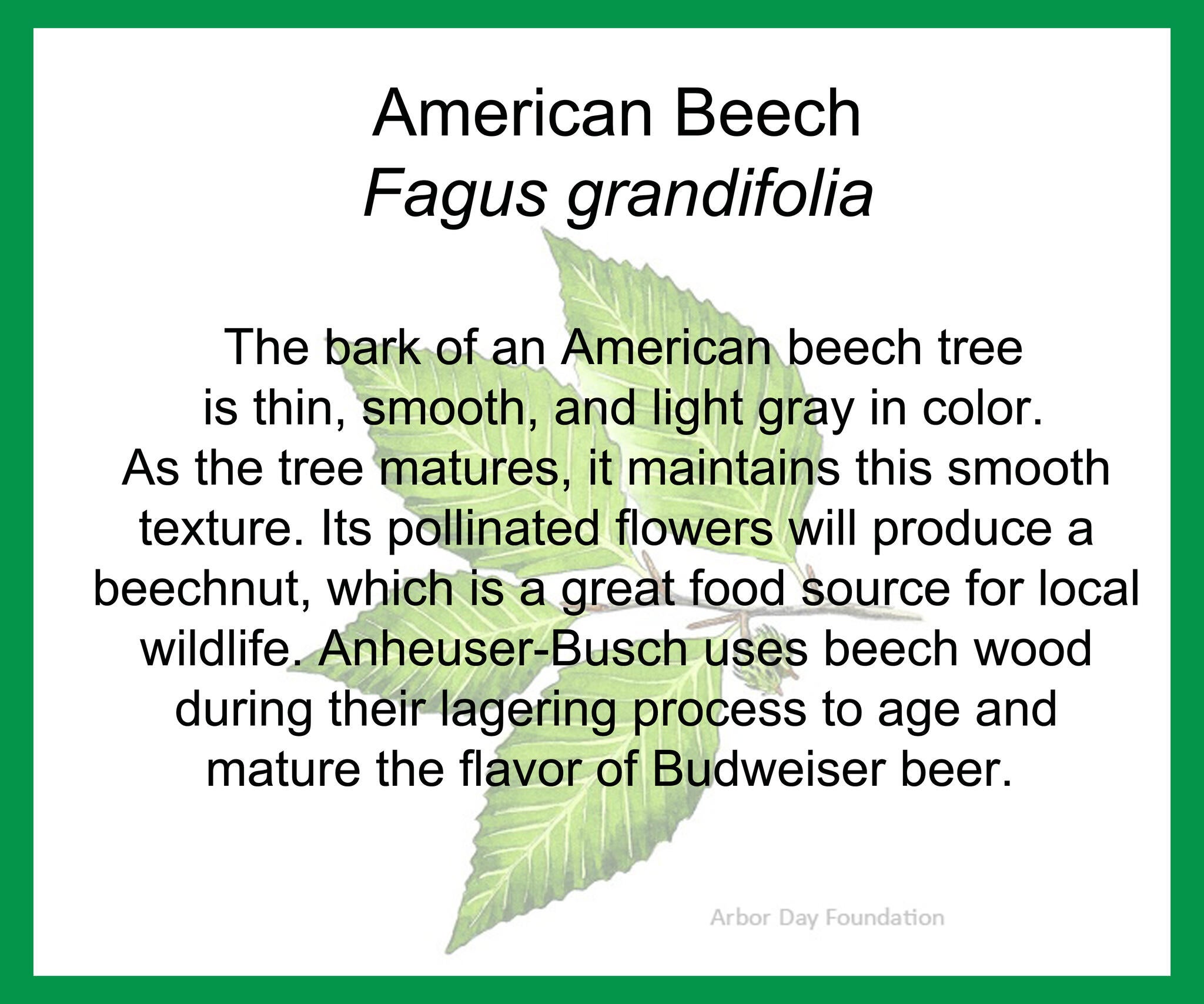This is an educational infographic provided by the Arbor Day Foundation on a white background with a green border. The central image features a semi-transparent twig with four elongated leaves that have pointed tips and serrated edges. Overlaid on the image in gray text is a detailed description. The header reads "American Beech, Fagus grandifolia." The accompanying paragraph describes the American beech tree's bark as thin, smooth, and light gray, maintaining its smooth texture as it matures. It explains that pollinated flowers of the tree produce beech nuts, which serve as an excellent food source for local wildlife. Additionally, it mentions that Anheuser-Busch uses beech wood during the lagering process to age and mature the flavor of Budweiser beer. There is a watermark in the lower right corner attributing the image to the Arbor Day Foundation. The leaves depicted are light green along the veins and darken towards the serrated tips.